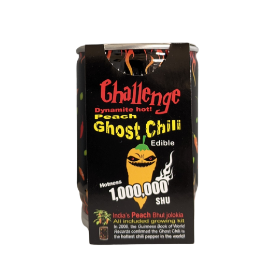In this photograph, we see an up-close image of a small, dark-colored (likely black) bag that contains hot peach ghost chili powder. The bag has a bold red caption reading "Challenge Dynamite Hot," emphasizing the extreme spiciness of the contents, which have a Scoville rating of 1 million. Prominently displayed on the bag is a graphic of an orange chili pepper character with black and red eyes, and a green stem-shaped hat. The pepper is diabolically smiling, enhancing the intense and possibly dangerous appeal of the product. Additionally, the words "Peach Ghost Chili" are written in yellow text, and there's a fine print warning about consuming the product safely. The background of the package is primarily black, making the vibrant text and the chili pepper character stand out dramatically. The bag features a silver rim at the top, suggesting it might be resealable.